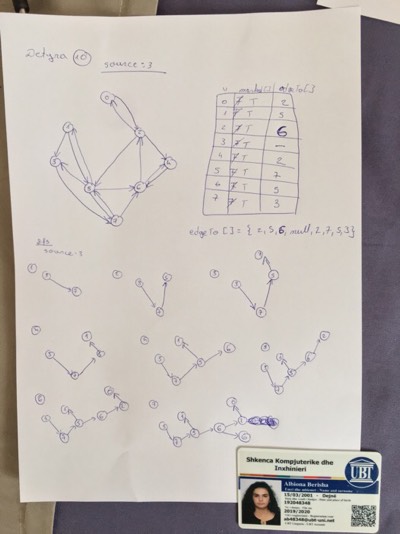This photograph captures a meticulously arranged scene featuring an 8½ by 11-inch piece of white paper. The paper is placed atop a closed blue notebook, which rests on a tabletop. In the upper left corner of the image, a pen is partially visible, hinting at recent use.

A key element in the bottom right corner is an identification card from an institution or company abbreviated as UBI. The card is fairly small, featuring a photograph of a woman on the left-hand side, some text likely in German, and a barcode, suggesting it is either an official ID or a membership card.

The white paper contains intricate blue pen sketches and writings, which resemble molecular or network diagrams. These consist of numerous circles connected by lines, each circle containing a small, often illegible number. The upper section of the paper features three rows of three circles, arranged somewhat like the letter 'H', all interlinked with lines, arrows, and numbers 3 and 4 prominently marked.

The bottom half of the sheet shows various groupings of circles ranging from three to six per cluster, depicting an increasing complexity in their connections. Each group is unique – some circles have multiple connections, while others have just one.

In the upper right corner of the paper, there's a neatly drawn rectangle divided into three columns. The first column lists numbers from 0 to 7, the second column contains an unrecognized symbol followed by a 'T,' and the third column lists the sequence: 2, 3, 6, blank, 2, 7, 5, 3. This chart likely provides a key to understanding the diagrams on the rest of the sheet.

This detailed caption offers a thorough description of the complex scene, highlighting its various elements and their potential significance.